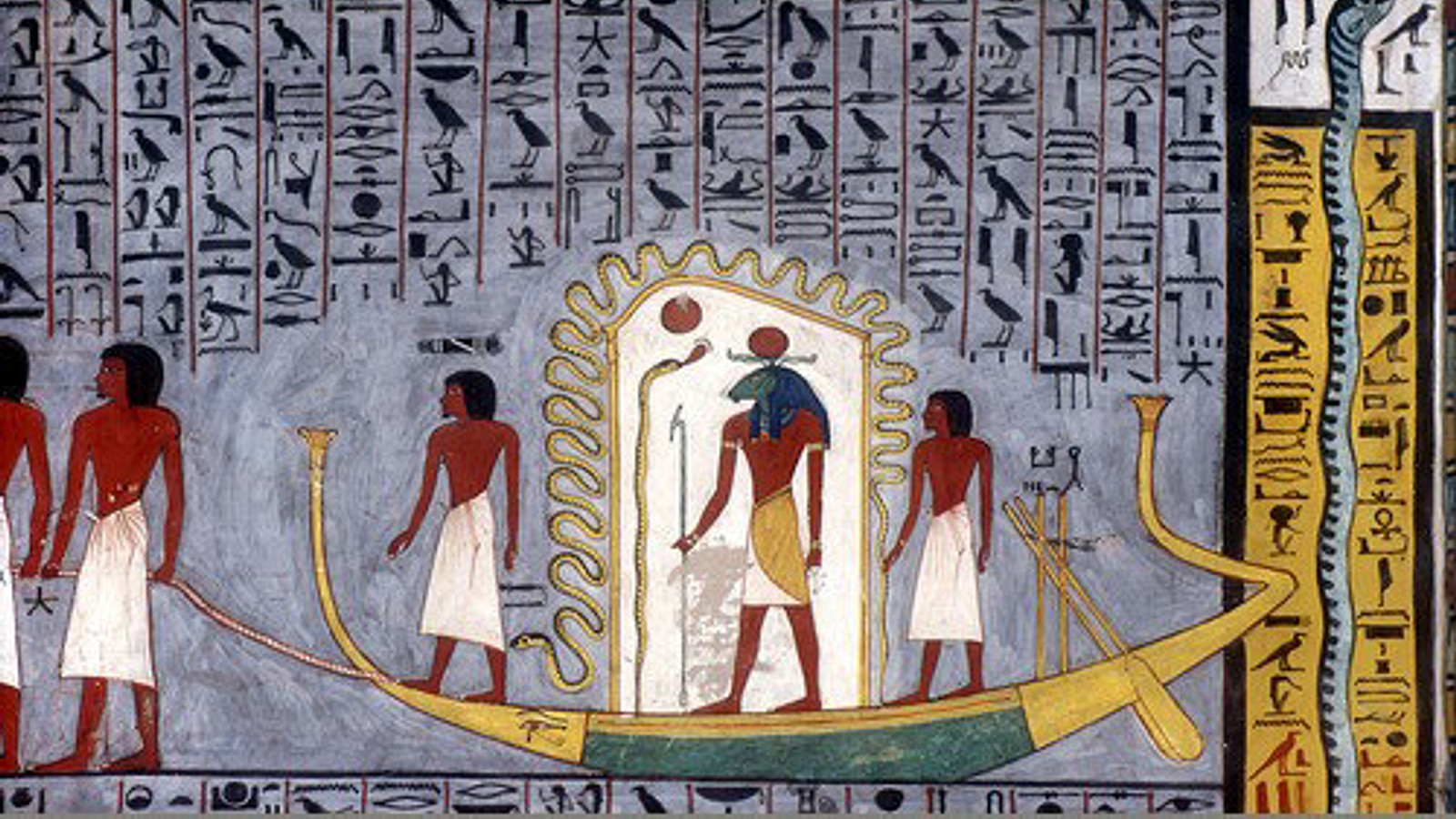The image is a detailed depiction of Egyptian art, reminiscent of what one might find adorning the walls of a pyramid. The background is a light bluish-gray with intricate hieroglyphs arranged in vertical lines across the top. Among the most frequent hieroglyphs, birds are prominently featured. Below, the scene transitions into a vivid tableau of five brown-skinned figures, adorned in white skirts. 

At the heart of the image is a golden boat with a green bottom, shaped like a canoe. On the boat, one man stands at the front and another at the back, both wearing white skirts. Between them, a figure, likely a deity, stands with a blue head and a circular red headdress, holding a staff. This figure's attire is a combination of white and gold. 

The boat is tethered by a rope held by two additional men on what seems to be land or a platform, similarly clad in white skirts. To the right, a golden box outlined in black contains more hieroglyphs and is intersected by a large black snake. The yellow and green color schemes of the boat and the detailed depictions of the figures, along with the hieroglyphs, create a narrative that is both rich in cultural symbolism and artistic detail.